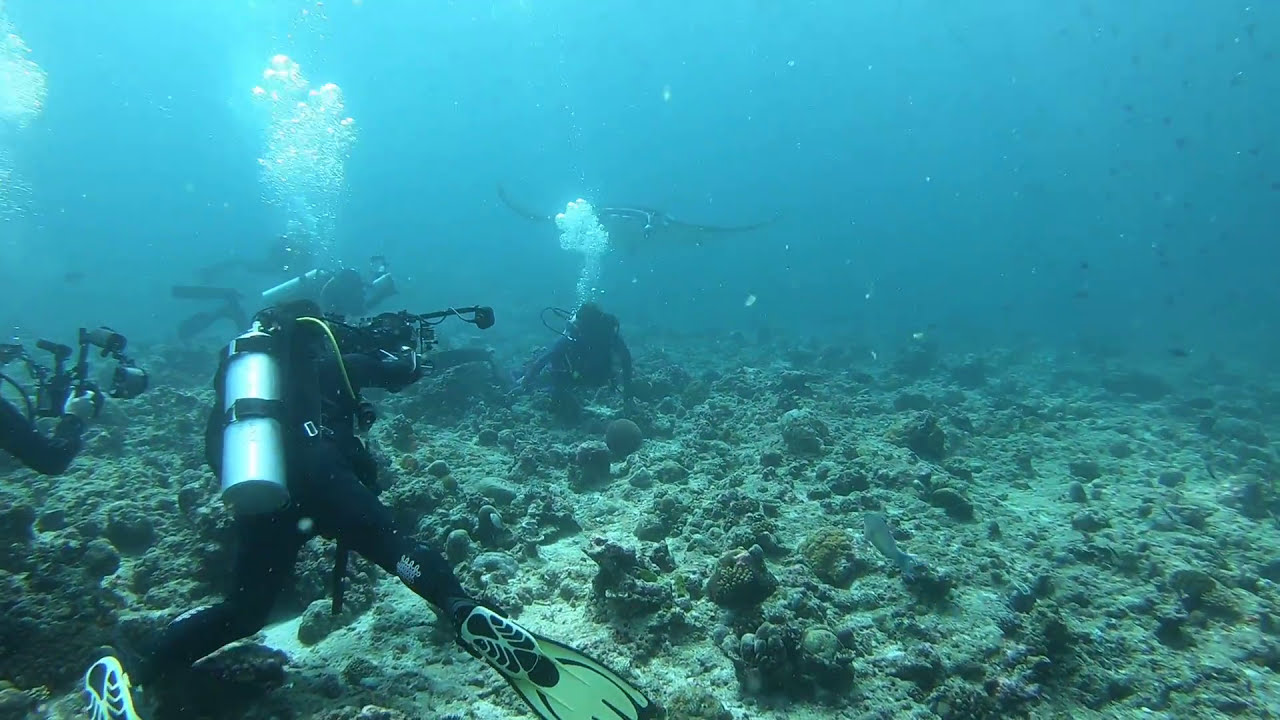In this detailed underwater scene, likely set in the ocean, there are five divers, each equipped with scuba outfits and oxygen tanks on their backs, exhaling bubbles from their breathing apparatuses. Three of these divers are positioning waterproof cameras, seemingly capturing a manta ray that gracefully swims in the center of the image. Beside them, small fish and possibly a tiny shark navigate the waters. Off to the right, a creature with long flippers, potentially a sea turtle, is visible. The ocean floor is a mosaic of light-colored sand, various corals, rocks, and marine plants, all enveloped by a blue-tinted ambiance. The diver in the forefront is notably outfitted with yellow and black fins, a black wetsuit, and a silver air tank, adding a splash of vivid color to this serene underwater tableau.